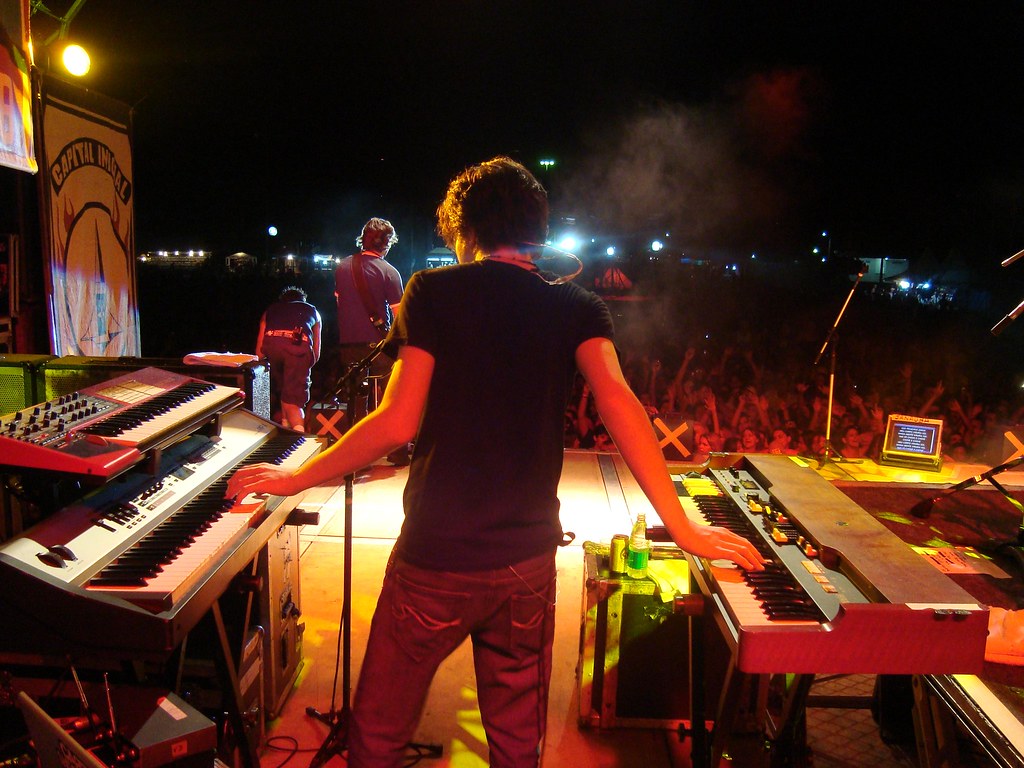This captivating photograph captures the electrifying atmosphere of a nighttime outdoor concert from a unique vantage point behind the keyboardist. The focus is on a young male musician with short, dark curly hair, dressed in a black t-shirt and blue jeans, skillfully playing two keyboards simultaneously. The one on his right features a distinctive red siding and black and white keys, while the setup on his left comprises a larger black keyboard with a silver panel and a smaller red keyboard positioned above it, possibly a Nord Lead.

The stage is set aglow with a mix of yellow and white lights, casting a warm, reddish hue over the musicians and the front rows of the enthusiastic crowd, whose raised hands seem to pulsate with the energy of the performance. To the left of the keyboardist, another band member in a blue t-shirt and pants carries a guitar, suggested by the visible strap, while a third performer, dressed in a blue shirt and shorts, leans towards the crowd, further engaging with the audience.

Additional stage details include various travel cases for equipment, microphone stands, and a small monitor displaying the song lyrics, although they are too distant to be read. Nearby, a beer bottle rests on a speaker, adding to the casual and immersive concert atmosphere. Beyond the stage, faint city lights twinkle against the black night sky, completing the scene of this dynamic live performance.